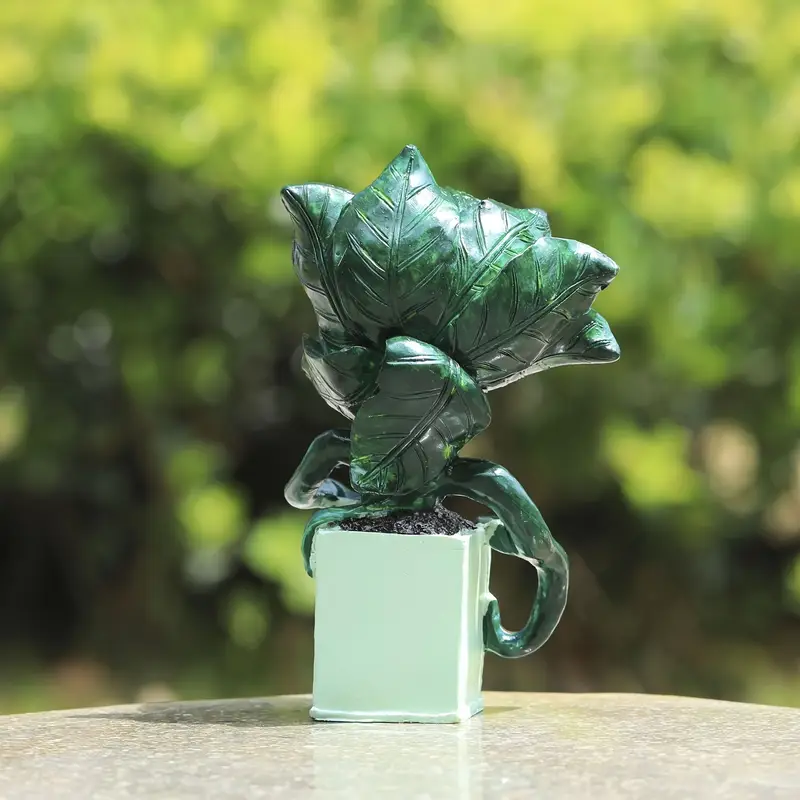The photograph captures a detailed ceramic sculpture of a plant set within a square, light green pot, highlighted by its intricate craftsmanship. The pot, square from above and rectangular from the front, contains what appears to be real soil, contrasting with the ceramic plant itself. The dark green leaves, some curling, flop down and are attached to the pot, revealing their sculpted nature by the matching paint at their tips. The leaves feature scratched patterns mimicking veins, adding to the realistic appearance. This meticulously crafted piece rests on a round table that seems to be made of stone, concrete, or metal, though only part of its surface is visible. Behind the sculpture, out-of-focus trees and foliage provide a blurred green background, emphasizing the sculpture’s details in the foreground. The overall presentation suggests portrait mode in photography, enhancing the distinction between the sharp foreground and the diffused natural backdrop.